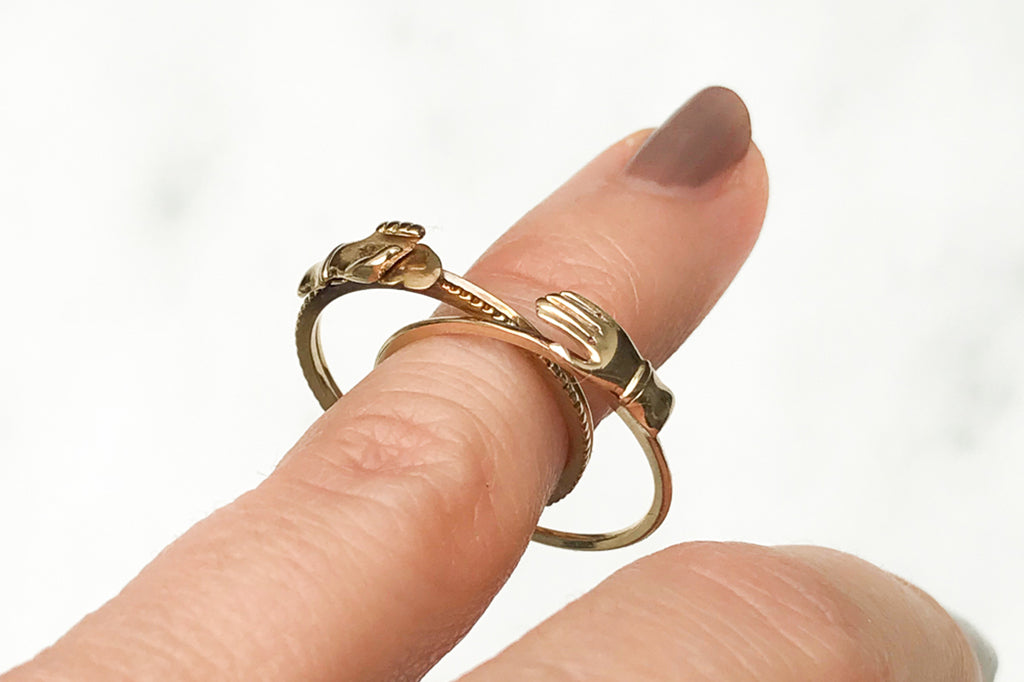This extremely close-up photograph captures two golden rings adorning the index finger of a woman's left hand against a white backdrop with subtle gray splotches. The focus of the image is on the two delicate, thin rings, situated just below the nail on the distal joint of the finger, giving the appearance that they are in the process of being worn and are slightly dangling. One of the rings features a detailed design motif resembling a gloved hand, while the second ring is a simple band, possibly with a subtle crown-like shape. The woman's finger boasts a well-manicured look with long nails painted in a light brown shade, revealing some growth at the base where the natural nail shows through. Only the section of the finger below the knuckle is visible, with the remaining finger bent out of sight.